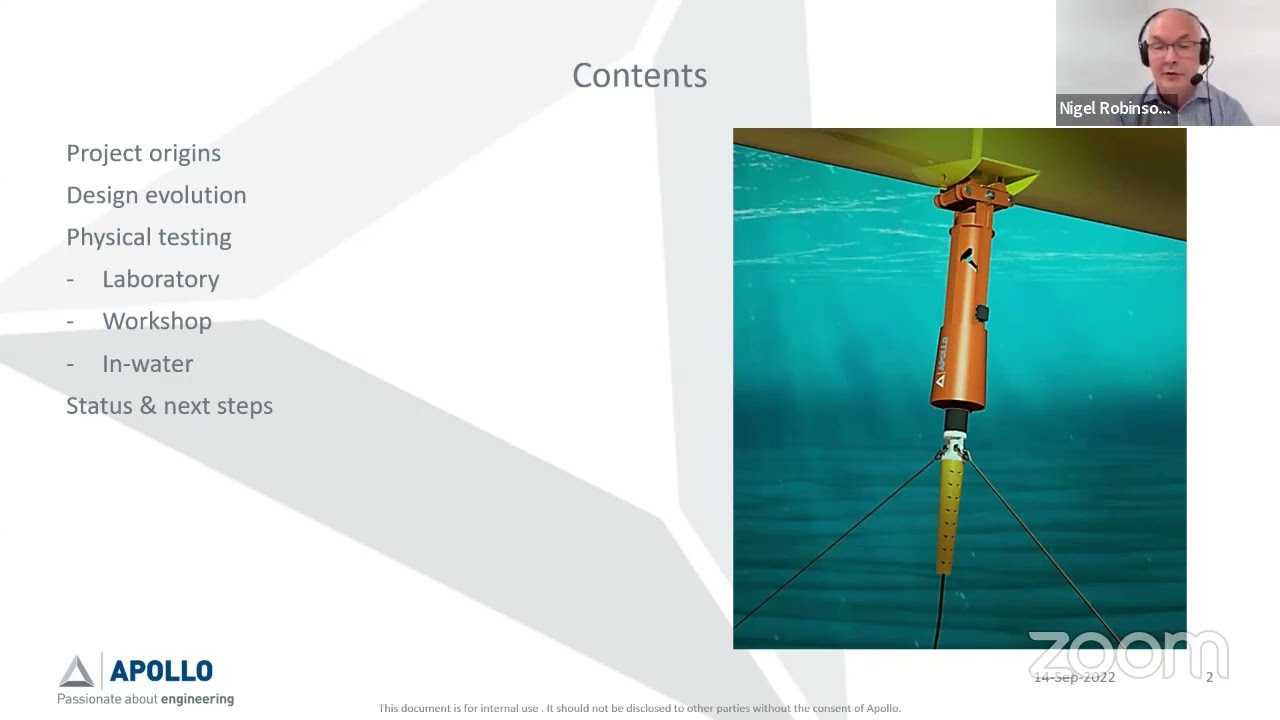The image is a detailed screenshot from a Zoom presentation meeting. At the center of the slide, the title "Contents" is displayed in light gray. Below this title, the slide lists various topics such as "Project Origin," "Design Evolution," "Physical Testing," followed by indented sub-topic "Laboratory," then "Workshop," "In Water," "Status," and "Next Steps." An additional text at the slide's bottom states, "This document is for internal usage, should not be disclosed to other parties without the consent of Apollo," dated 14 SEP 2022. In the bottom left is the Apollo logo, with a vertical blue text "Apollo" and underneath it reads "passionate about engineering."

On the right side of the slide, there is a detailed computer graphic showing an underwater device. This device features an orange pole with a top bracket connected to a surface, tapering down to a segment with cables branching in three directions forming a triangular shape.

In the top right corner is a small video feed of the presenter, Nigel Robinson. He appears bald, with glasses, wearing a headset and a microphone, donned in a blue button-down shirt. Alongside his image, the Zoom overlay displays, confirming the video call. The transparent text overlay slightly shows "Nigel Robinson" along with some text cut off by a rectangle. The overall scene encapsulates a professional engineering presentation facilitated virtually via Zoom.